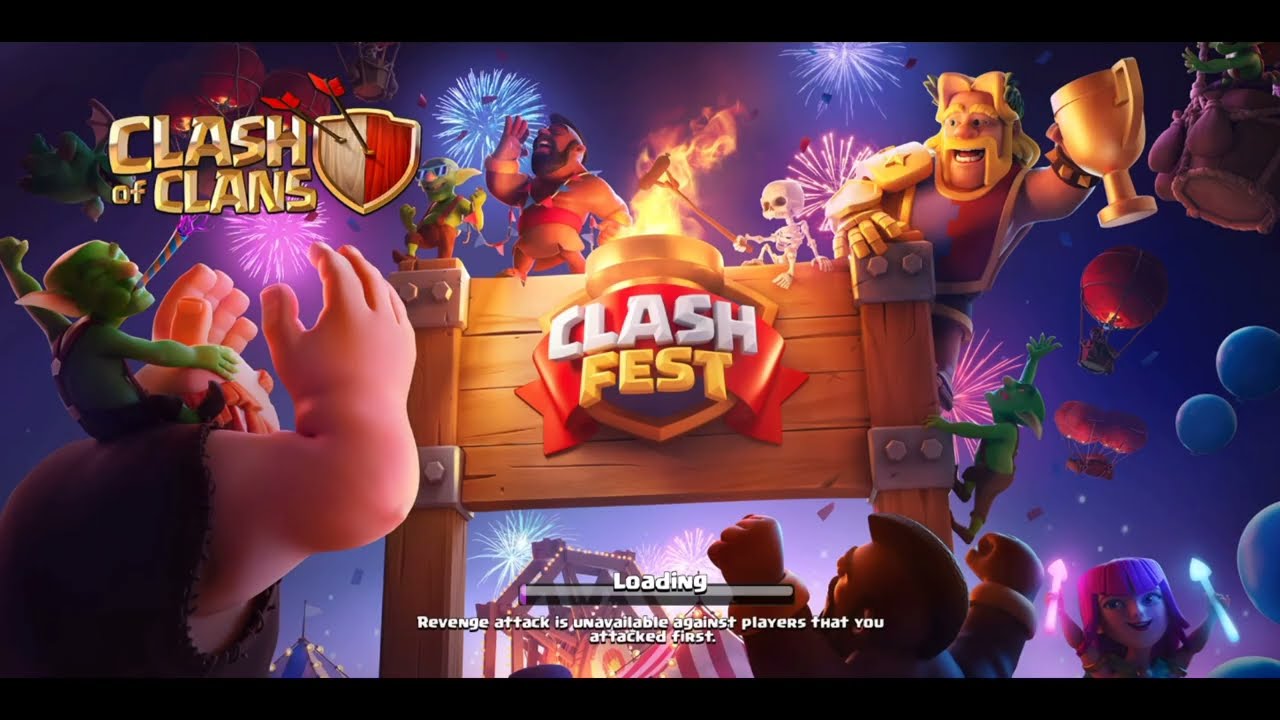The captivating image showcases a vibrant loading screen from the popular video game Clash of Clans. In the upper left corner, the game's title is emblazoned in gold, accompanied by its iconic shield logo, which features a light brown and red split background with two arrows embedded in it. Dominating the center is a wooden archway adorned with a red ribbon that announces "Clashfest." Surrounding the archway are various animated characters from the game. Notably, a large character with exaggerated arms and hands, wearing a green mini version of himself on his shoulder, stands with his back to the viewer. Other characters include a Hercules-like figure hoisting a gold trophy, a skeleton who appears to be barbecuing, and cheerful spectators gathered around. Fireworks light up the sky in the background, adding to the festive atmosphere. At the bottom center, a loading bar, filled with gray, is underscored by white text stating "Revenge Attack is unavailable." The scene is a lively depiction of excitement and celebration, characteristic of Clash of Clans events.